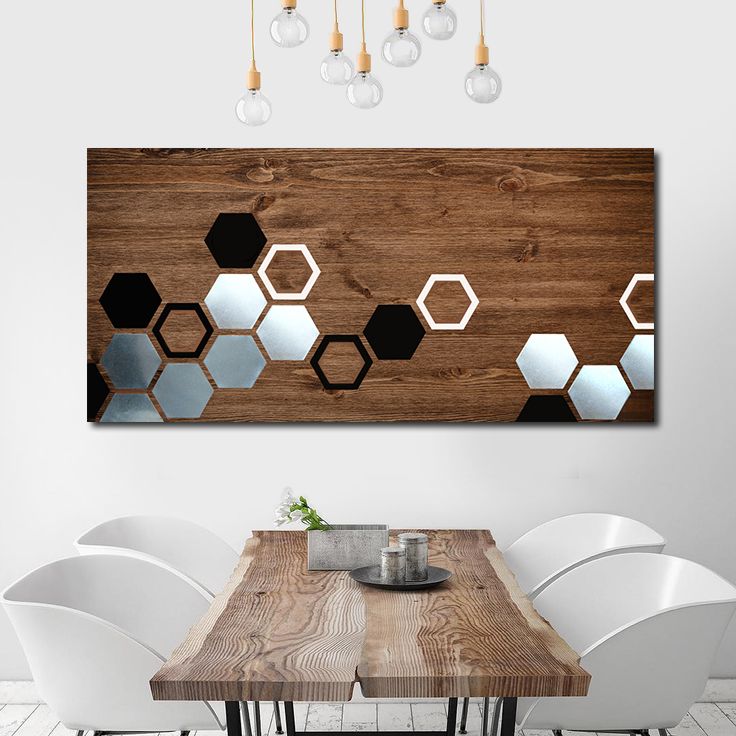The image depicts a modern, stylish dining area. The background features a light gray or white wall adorned with a rectangular piece of abstract art that appears to be set on a wooden canvas. The artwork consists of scattered hexagons in black, white, and silver, some solid and some outlined, adding a geometric flair to the space. Suspended from the ceiling are elegant Edison bulb lights hanging from long golden stems, casting a warm glow over the room. Below the artwork stands a robust wooden dining table with black legs, seemingly crafted from a single tree trunk, surrounded by four sleek, white, scoop-shaped modern chairs. Upon the table sits a metal plate holding metal canisters and a small gray metal box containing floral greenery, contributing to the room's sophisticated yet cozy ambiance.